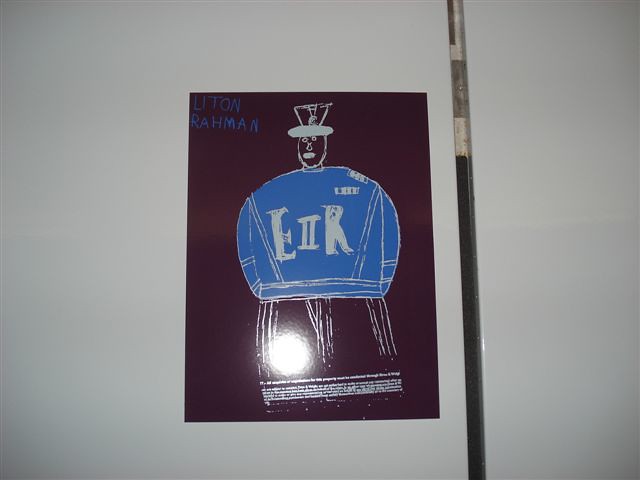The image features a square poster hanging on a white wall, displaying a child-like drawing of a male figure. The background of the poster is predominantly black, while the main colors within the drawing are blue, tan, and brown. The top segment of the poster prominently displays the name "Latan Rahman" in blue letters. The drawing itself presents a somewhat detailed stick figure, resembling a caricature with a disproportionately large midsection, suggesting a heavy-set person. The figure wears a navy blue or purple sweatshirt emblazoned with the fragmented text "E2R" or "E-R" in white. The figure also sports a hat, described variably as a top hat or a baseball hat. The pants are depicted as very wide, colored black with white outlines. The overall artistic style appears to be rudimentary, as if drawn by a young child, and could be an illustration from a book or a simple sketch. The white part of the wall also features a long, black stick with sections alternating in white and gray, which leans against the wall near the poster.